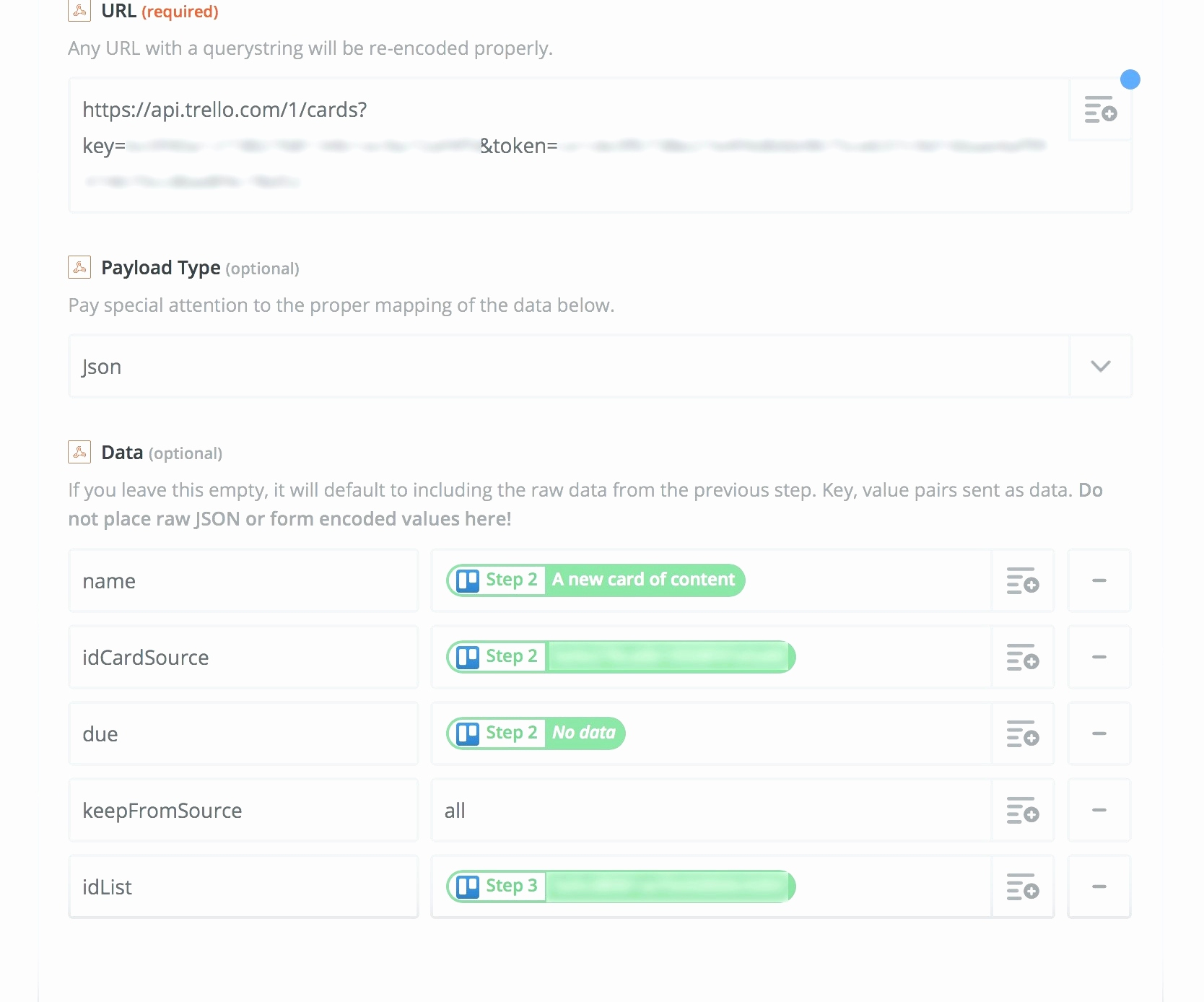The image displays a white background featuring a section of a UI form prominently related to API calls. In the upper-left corner, it reads "URL" with the text "(required)" in red indicating a mandatory field. Below that, there's a note in black text: "Any URL with a query string will be re-encoded properly."

The next line shows an example API endpoint: "HTTPS://API.trello.com/1/cards?" followed by "key=" and an anonymized (whited-out) API key, then "token=" followed by another whited-out section.

Further down, under "Payload Type" in black with "(optional)" in gray, a note advises to "pay special attention to the proper mapping of the data below." There's a shaded gray box labeled "JSON" with a right-pointing arrow, presumably for expanding.

Following that, it states "Data" in black and "(optional)" in gray. An informative note reads: "If you leave this empty, it will default to including the raw data from the previous step. Key-value pairs set as data should not include raw JSON or form-encoded values here."

Below this, the label "Name" is presented atop an outlined banner reading "Step 2" in the center. To the right, in a green banner with white text, it says "A new card of content." The far-right section features four small purple lines and a purple box with a minus sign.

The next section includes "ID Card Source" associated with "Step 2." The green text within this step is whited out, flanked by four small horizontal lines and a minus sign in purple.

Subsequently, the label "Do" appears, marked "Step 2" with a small green banner saying "No data," leading over to the same four purple lines and minus sign setup.

For "Keep From Source," the middle reads "All" with the same layout on the right.

Finally, "ID List" links to "Step 3," again with whited-out content in the green banner on the right, alongside the purple lines and minus sign. 

The overall composition suggests a highly structured form for managing API calls and data mappings, with key sections editable for user data inputs or configurations.